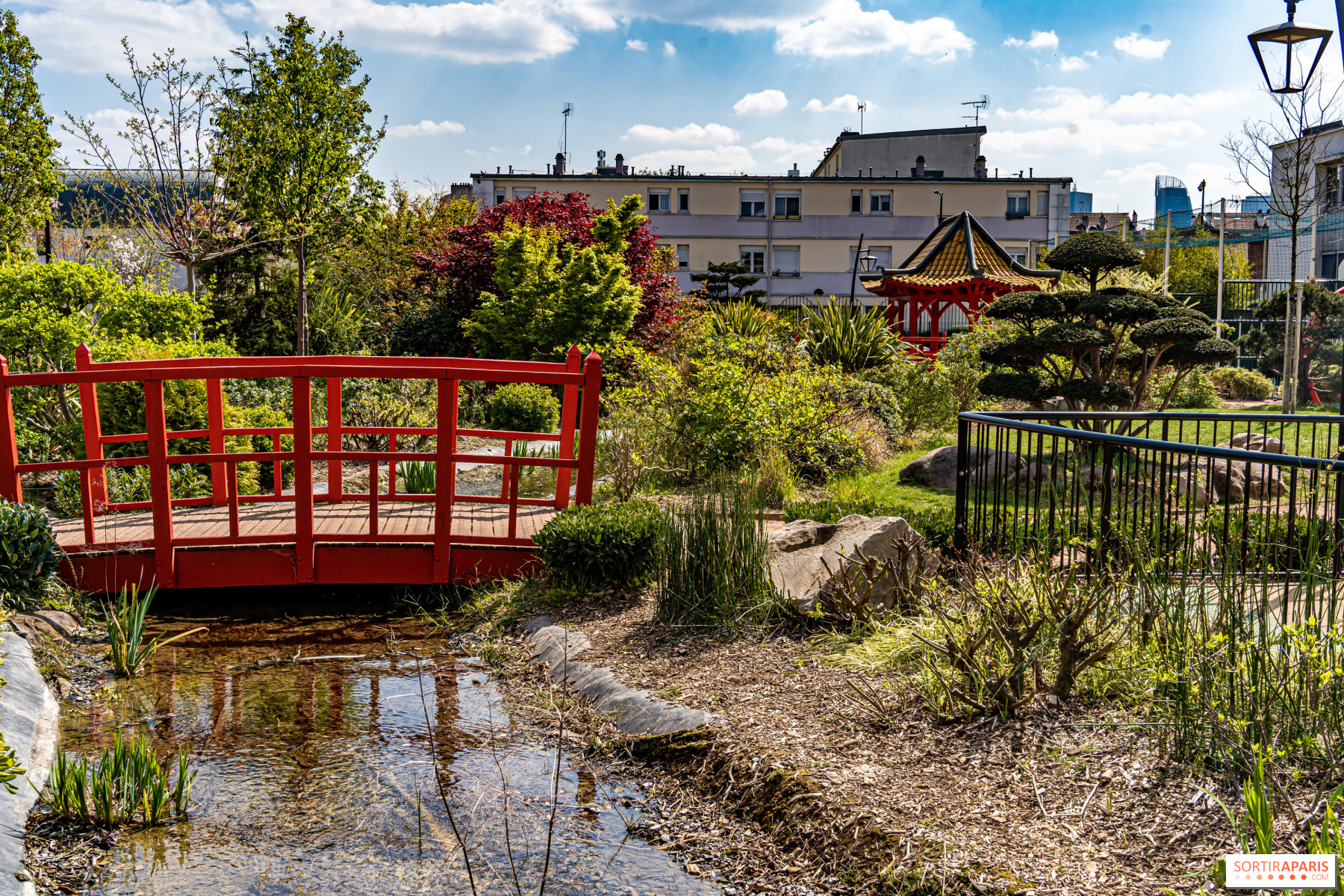The image depicts a serene, well-maintained garden or park nestled within an urban setting, characterized by low apartment buildings in the background. Dominating the foreground is a slightly arched, red-painted bridge that crosses a small, possibly artificial stream lined with reeds and various bushes. To the right of the bridge, a waist-high steel fence marks the boundary of the garden area. The ground is thoughtfully mulched, supporting a variety of trees and shrubs, mostly green, but including some with brown or red foliage. A concrete path can be seen just behind the bridge, and in the background, a structure with a pagoda-style roof, possibly covering a picnic table, adds a touch of traditional architectural charm to the scene. The setting is further enriched by a glass lantern peeking from the upper right corner and the clear blue sky with scattered clouds overhead.